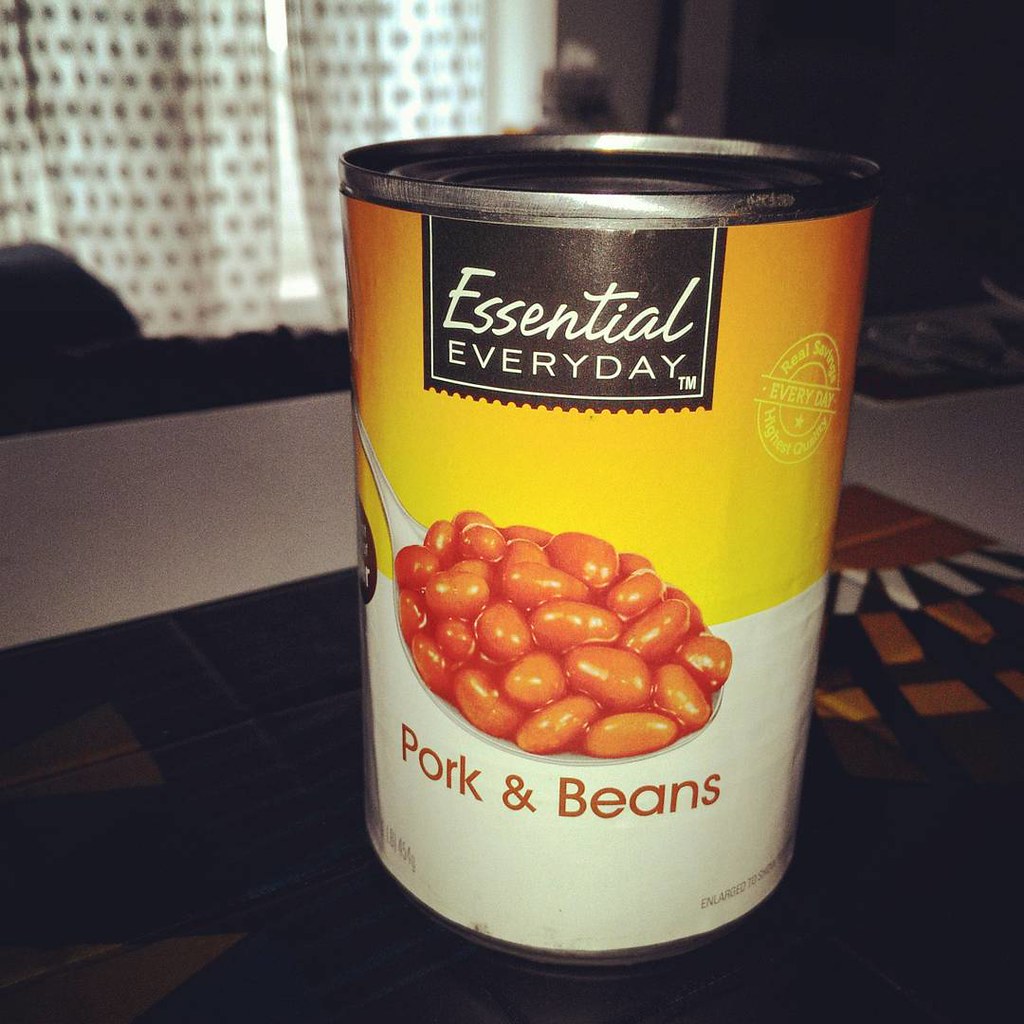This is a detailed photograph of a standard-sized can of Essential Everyday Pork and Beans, captured in a dimly lit environment with flash. The can sits on a kitchen counter, which appears white with black tile inlay, next to a dark placemat. The label of the can is divided into two halves: the top being yellow and the bottom white. The brand name, Essential Everyday, is displayed on a black, postage-stamp-like label at the top, with "ESSENTIAL" in white handwriting and "EVERYDAY" in Arial uppercase font with a trademark indicator beside it. Below this, there is a spoonful of pork and beans pictured in a rich sauce, and the product name “Pork and Beans” is written in red lettering. Additional labeling includes a white circular stamp indicating "Real Savings and Highest Quality Everyday." The surroundings include a white curtain with black spots drawn over a window, allowing some daylight to peek through, enhancing the details of the countertop and the can’s vibrant label among the otherwise dark interior, suggesting the photo was taken at night or in low interior lighting.